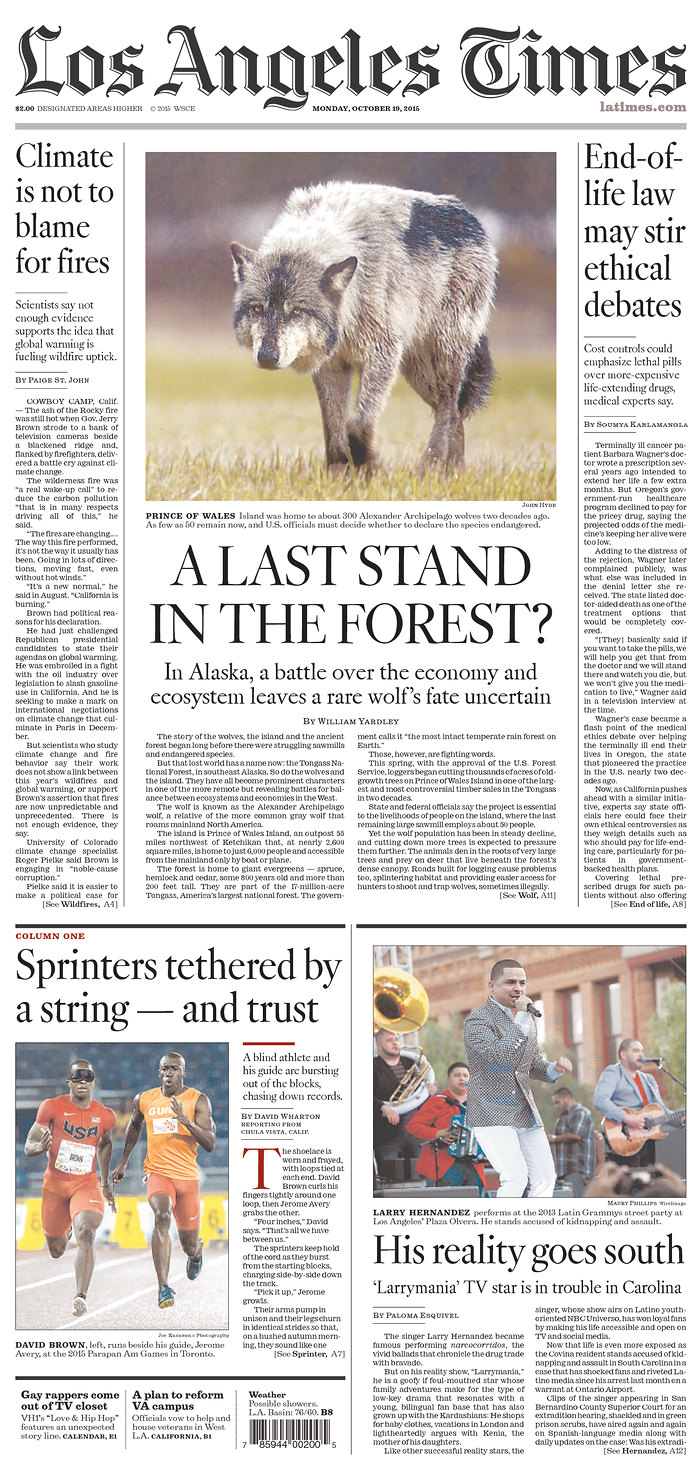This image is a photograph of the front page of the Los Angeles Times, captured from the October 19, 2015 edition. The newspaper is priced at $2.00, with specific locations having a higher price, as noted at the top. The masthead features "Los Angeles Times" in bold, stylishly-lined font, accompanied by the website "latimes.com."

Prominently centered on the page is the headline: "A Last Stand in the Forest." This lead article discusses a battle over the economy and ecosystem in Alaska, focusing on the uncertain future of a rare wolf species. Dominating the page is a large photograph of an Alexander Archipelago wolf, showcasing its predominantly black, gray, and white fur as it gazes pensively towards the camera. The caption below the image reads: "Prince of Wales Island was home to about 300 Alexander Archipelago wolves two decades ago; as few as 50 remain now and U.S. officials must decide whether to declare the species endangered."

To the left, another headline states, "Climate Not to Blame for Fires," while to the right, an article titled, "End-of-Life Law May Stir Ethical Debates," indicates a discussion on contentious legislative changes. Additional articles and images populate the lower section of the page, providing further news and insights. The entire page is under copyright 2015 by WSCE.